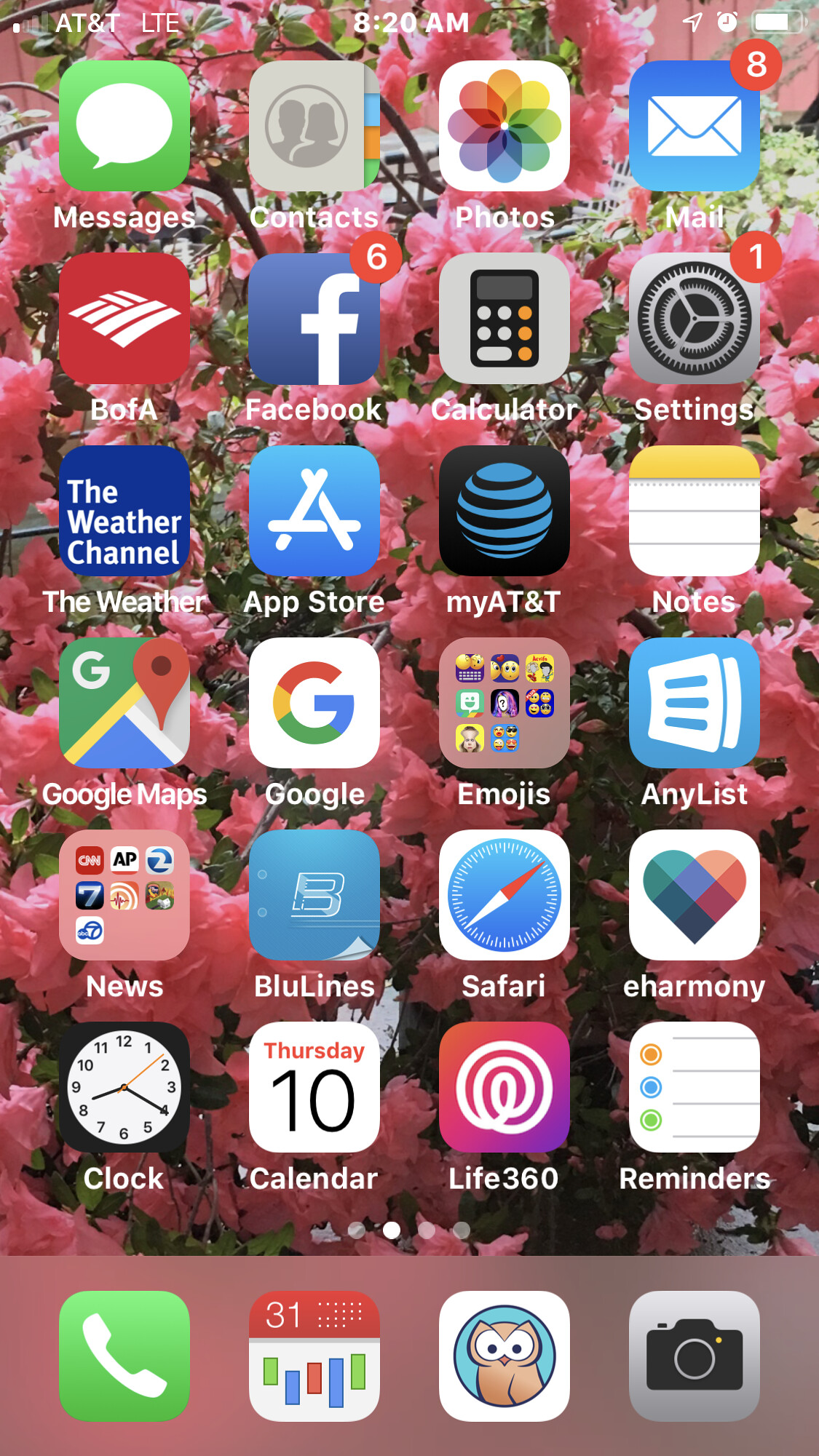This tall, rectangular image portrays a digital display reminiscent of an app directory on a computer or mobile phone screen. Arranged in a grid format, the image features four app icons across and seven down, totaling twenty-eight apps. Each app icon showcases vibrant colors and intricate details, making the overall composition lively and engaging. The background features a dense layer of vivid pink cherry blossoms, adding an extra element of visual complexity to the scene. The juxtaposition of the colorful, informative app icons against the bustling, floral backdrop creates a striking and busy aesthetic. Many of the app icons appear familiar, suggesting commonly used applications, evoking the sense of navigating through an actual apps or settings page on a digital device.